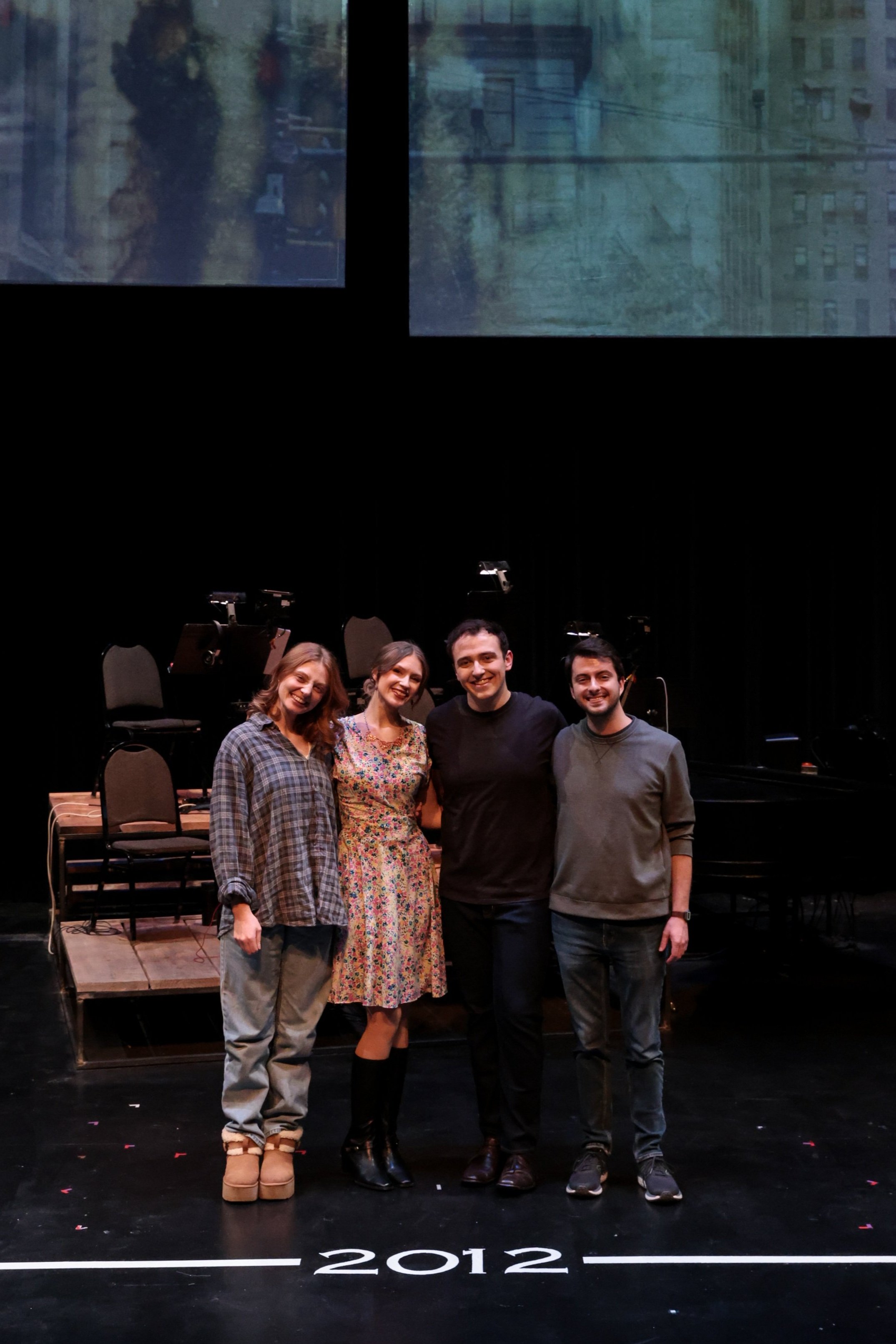This color photograph captures four people standing on a stage, whose black floor contrasts with the wooden platform and black metal chairs positioned behind them. The image is in portrait orientation, with the year "2012" displayed in white text at the bottom. Two large white banners hang from the ceiling in the background, framing the scene. The four individuals, who appear to be in their 30s, stand closely together, with their hands behind each other's backs, suggesting camaraderie possibly following a performance.

On the far left stands a woman in a casual outfit, consisting of a blue bikini top layered with a green plaid checkered button-up shirt, light blue jeans, and brown Ugg-like boots with platforms. Next to her, a woman wears a knee-length dress adorned with blue, pink, and green polka dots, complemented by tall black leather boots.

To the right of the women, a man in a black shirt, dark jeans, and black shoes stands. Completing the lineup on the extreme right is another man dressed in a gray sweatshirt and blue jeans. The casual attire of both men and the informal setting suggest a relaxed, friendly atmosphere. The entire group, composed of two women and two men, all Caucasian, face forward, capturing a moment of unity and casual comfort.